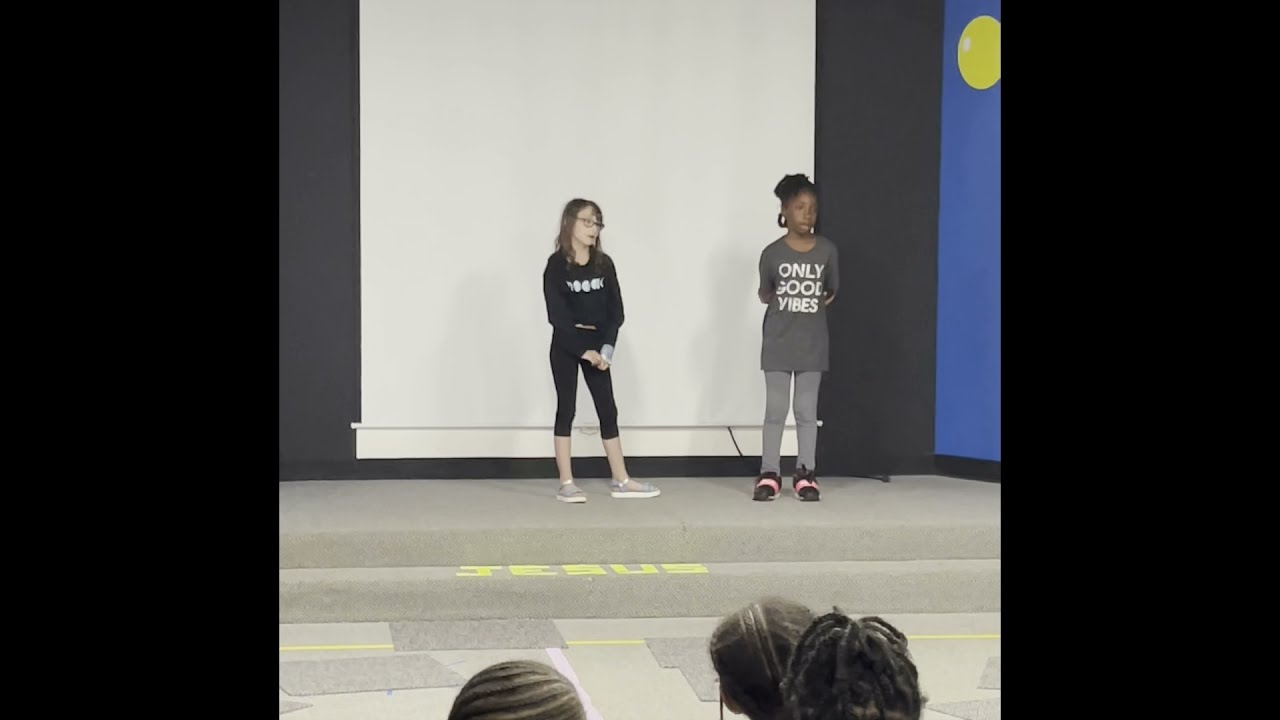This full-color photograph, taken indoors, captures a performance on a two-step elevated stage. The left and right edges of the horizontally rectangular image are framed by thick black borders. Center stage, two young girls stand in front of a large white projection screen. The shorter girl, on the left, is Caucasian with long brown hair, glasses, a black long-sleeve shirt, and black capri leggings that end just below her knees, paired with gray sneakers. The taller girl, on the right, is African American, possibly in her early teens, adorned with earrings, and dressed in a dark gray T-shirt that reads "ONLY GOOD VIBES" in large white letters, along with matching gray leggings and black shoes. Behind them, a blue wall with a yellow circle at the top is partially visible. The word "JESUS" is prominently displayed on the first stair in bright lime green tape, suggesting a religious context, possibly a school talent show. In the foreground, the tops of three young African American children's heads are visible, indicating an audience attentively watching the scene.